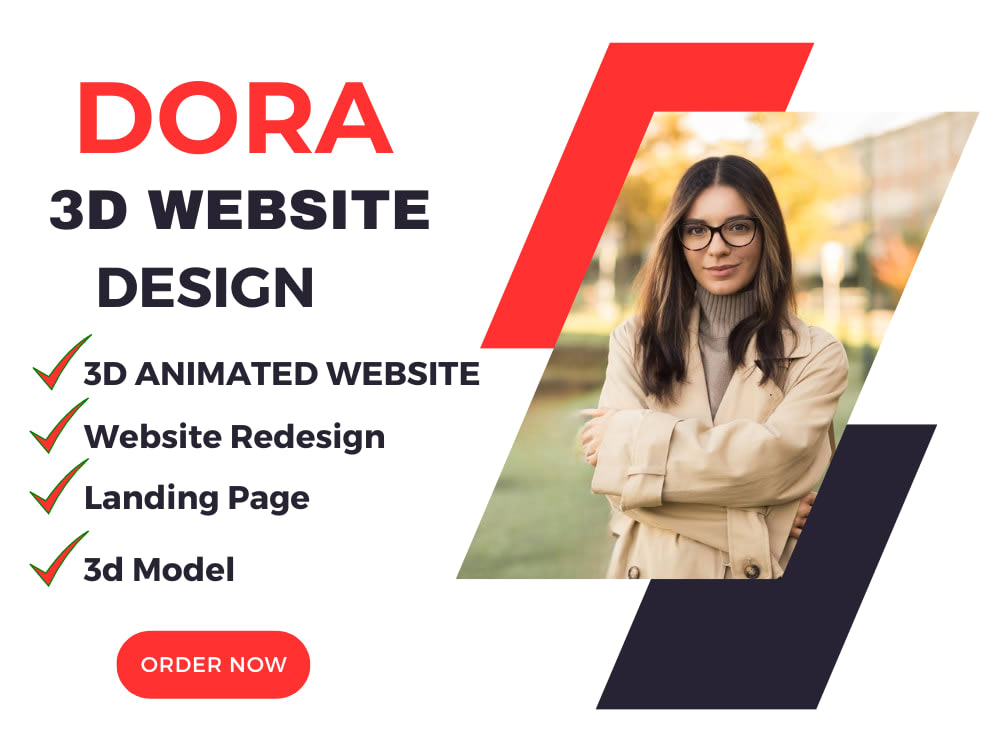This image features a white background with a detailed advertisement for a 3D website design service. On the left side of the image, the heading "Dora 3D Website Design" is prominently displayed, with "Dora" written in red and "3D Website Design" in black. Below the heading, four bulleted points with corresponding colorful check marks are listed in black text: "3D Animated Website," "Website Redesign," "Landing Page," and "3D Model." At the bottom, there is a red oval or rounded rectangle button that reads "Order Now."

On the right side of the image, there is a photograph of a Caucasian woman with long, brown hair and black glasses. She is standing with her arms folded in front of her chest and is looking directly into the camera. She is wearing a light tan jacket with buttons over a gray turtleneck. The background behind the woman is slightly blurred, suggesting an outdoor setting with trees, buildings, and sky visible. Above her are abstract red and black rectangles that complement the overall design of the ad.